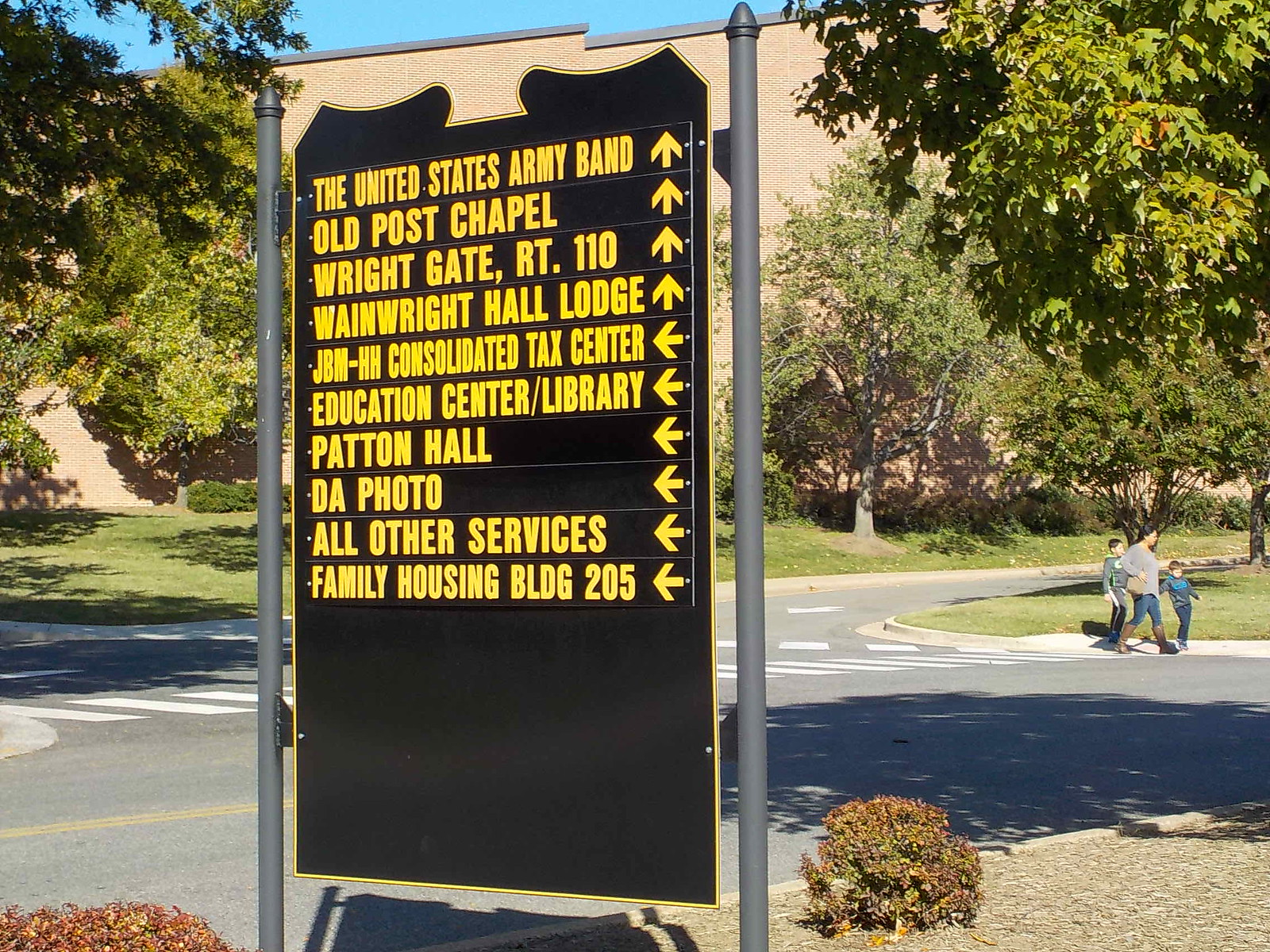This is a daytime photograph of a directional sign situated in or near a parking lot, with a clear blue sky overhead. The sign is suspended between two tall gray metal posts and features a long, rectangular black panel with a blue border and a designed pattern shape at the top. The sign is adorned with large yellow capital letters and arrows indicating various directions. The inscriptions read: "United States Army Band" with an arrow pointing up; "Old Post Chapel" with an arrow pointing up; "Wright Gate, Wright 110" with an arrow pointing up; "Wainwright Hall Lodge" with an arrow pointing up; "JBM-HH Consolidated Tax Center" with an arrow pointing left; "Education Center/Library" with an arrow pointing left; "Patton Hall" with an arrow pointing left; "DA Photo" with an arrow pointing left; "All Other Services" with an arrow pointing left; and "Family Housing Building 205" with an arrow pointing left.

The background features a mix of grassy areas, trees, and bushes, with a large brown brick building seen in the far distance. A walkable and motorable road strip is visible, along with a pedestrian crossing and a curb in the foreground. On the right side towards the middle, a lady is walking with two children on a sidewalk, surrounded by small plants and dirt patches. The overall scene is bright and well-illuminated by sunlight.